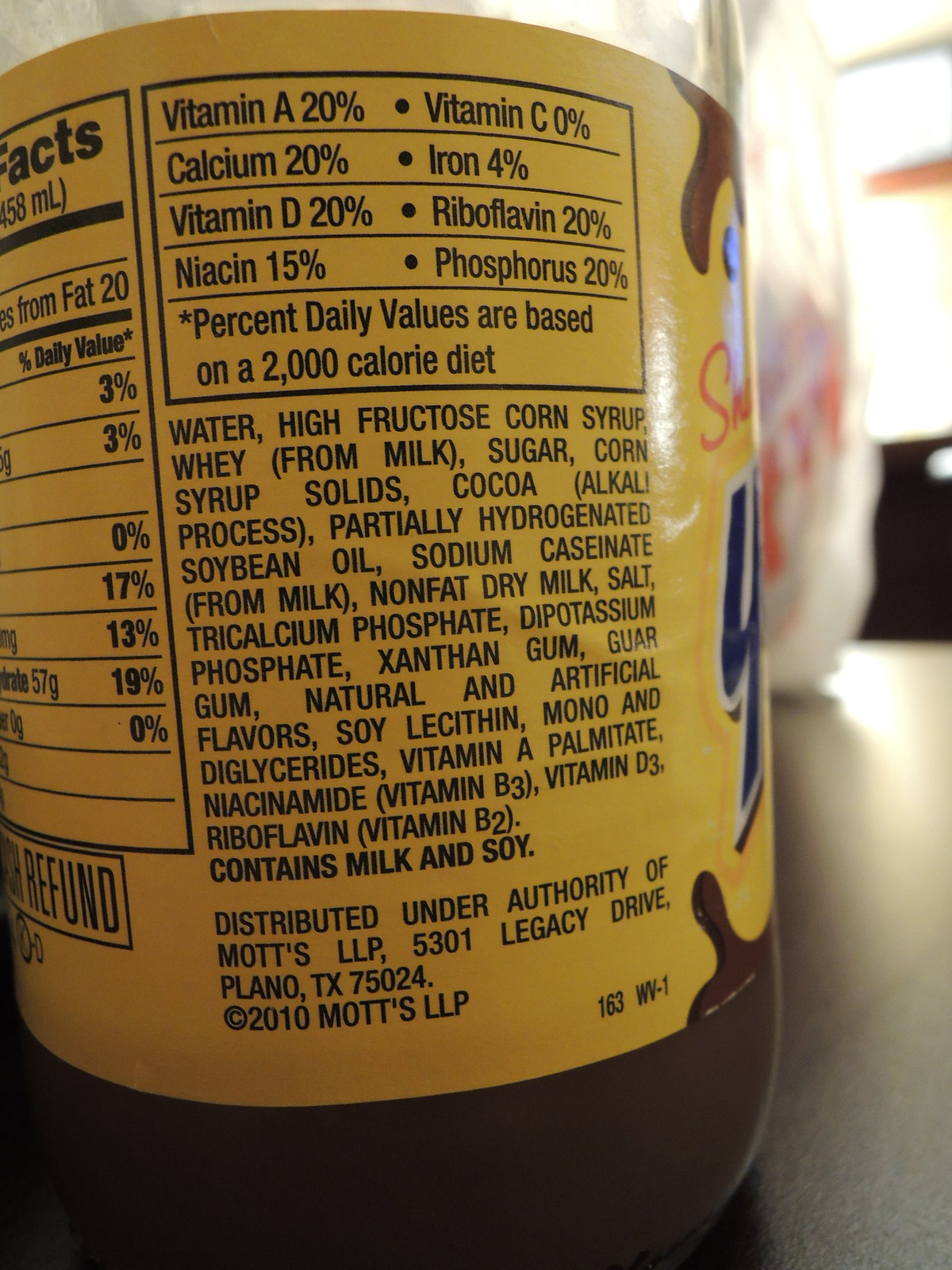This image depicts the back panel of a YooHoo chocolate drink bottle. The bottle features a yellow label on a clear container. A small amount of the YooHoo beverage is visible at the bottom, just beneath the label, while the top portion of the bottle remains empty. The label prominently displays nutrition information and ingredients. Despite seeing the back of the bottle, the iconic "Y" from YooHoo is partially visible on the side.

The yellow label is detailed with black text and black boxes. Notably, some text on the right side of the nutritional facts table is cut off. Visible details include "Calories from Fat: 20" and several percentage values of the daily intake: 3%, 3%, 0%, 17%, 13%, 19%, and 0%. Below these values, there is a barcode.

To the left of the barcode, another label lists specific nutritional information: Vitamin A (20%), Vitamin C (0%), Calcium (20%), Iron (4%), Vitamin D (20%), Riboflavin (20%), Niacin (15%), and Phosphorus (20%). It states that the percent daily values are based on a 2,000-calorie diet.

Further down, the label includes a comprehensive list of ingredients and the information, "Distributed under the authority of Mott's LLP, 5301 Legacy Drive, Plano, Texas, 75024. ©2010 Mott's."

In the background, part of the counter where the YooHoo bottle is sitting is visible, along with a window in the top left corner, which allows natural light to filter into the scene.